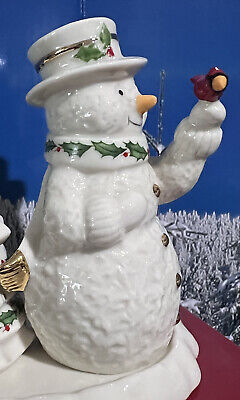The image showcases a shiny, white snowman figurine, likely made of porcelain, serving as festive Christmas decor inside a home. The snowman is standing on a white porcelain plate, set against a dark blue wall backdrop. Behind it, a Christmas tree or greenery dusted with artificial snow adds a seasonal touch. The snowman is oriented in profile, facing to the right, with one visible eye and an orange nose. It wears a white top hat adorned with holly and features a scarf with matching holly leaves. On its left hand, which is extended upwards, perches a red cardinal with a gold beak. The snowman's right arm rests by its side, and three dark buttons line the front of its belly. The detailed ornaments and festive elements make it a charming piece reminiscent of traditional Christmas decorations often seen in cozy family homes.